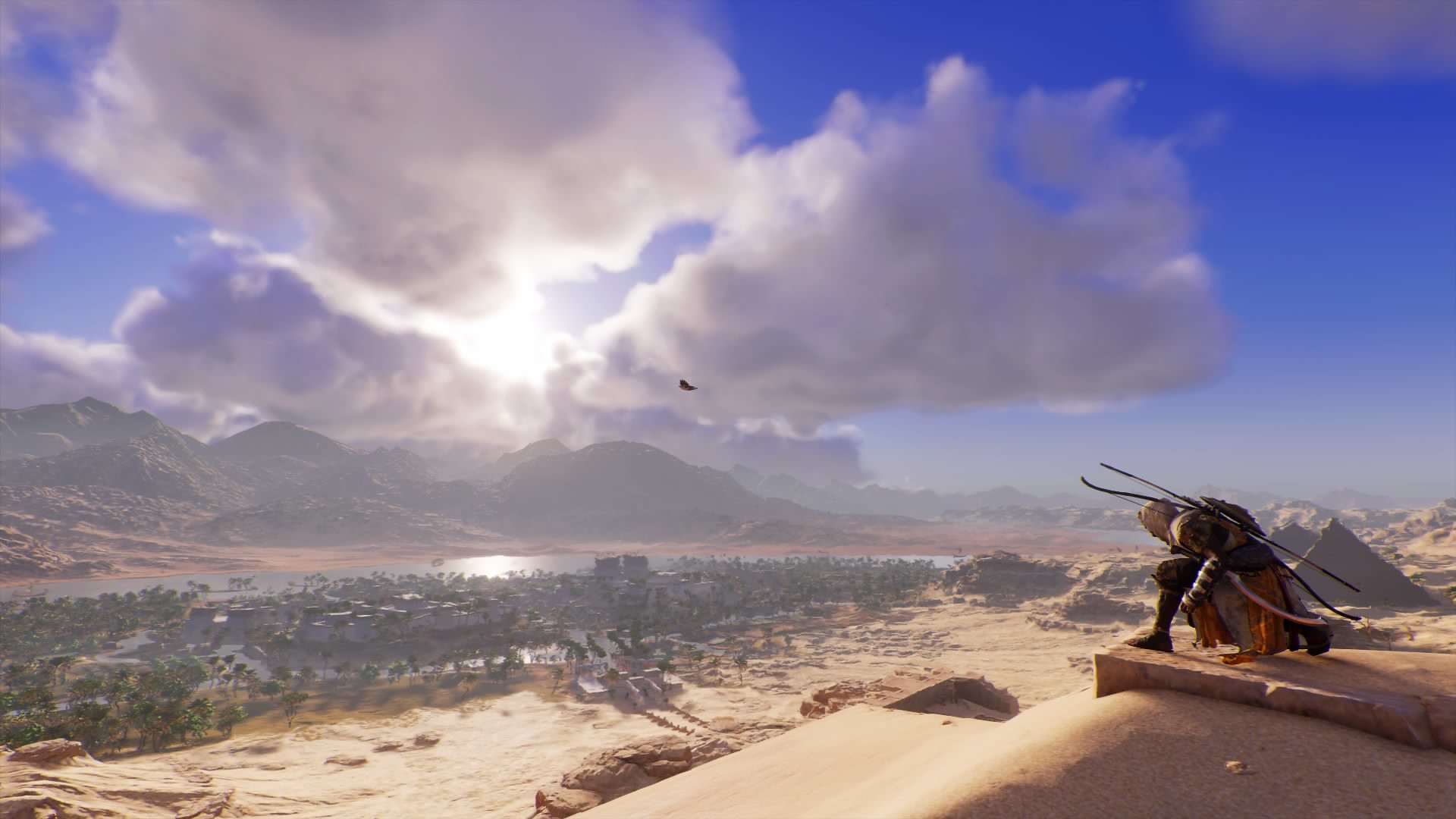In a computer-generated or animated image, a lone figure kneels on a dusty, sandy hillside in the middle of a vast desert, clad in a detailed military uniform that includes large brown boots and a beige hood. Across the person's back are imposing, long weapons—one of which appears to be a bow or crossbow, while another could be a sword. An orangey-red sash or belt is wrapped around their waist. The scene is illuminated by a bright, sunny sky dotted with some clouds, with the sun's rays beaming through. 

Below, a small city rests in a valley near water, under siege, with numerous figures embroiled in battle. Surrounding this valley, the landscape features a mountain range to the left, blending into the clouded horizon, and two distinct triangular pyramids to the right. The entire scene captures a sense of looming conflict and desolation under the clear blue sky, with the dark, tumultuous city contrasting sharply against the sandy, sunlit desert.